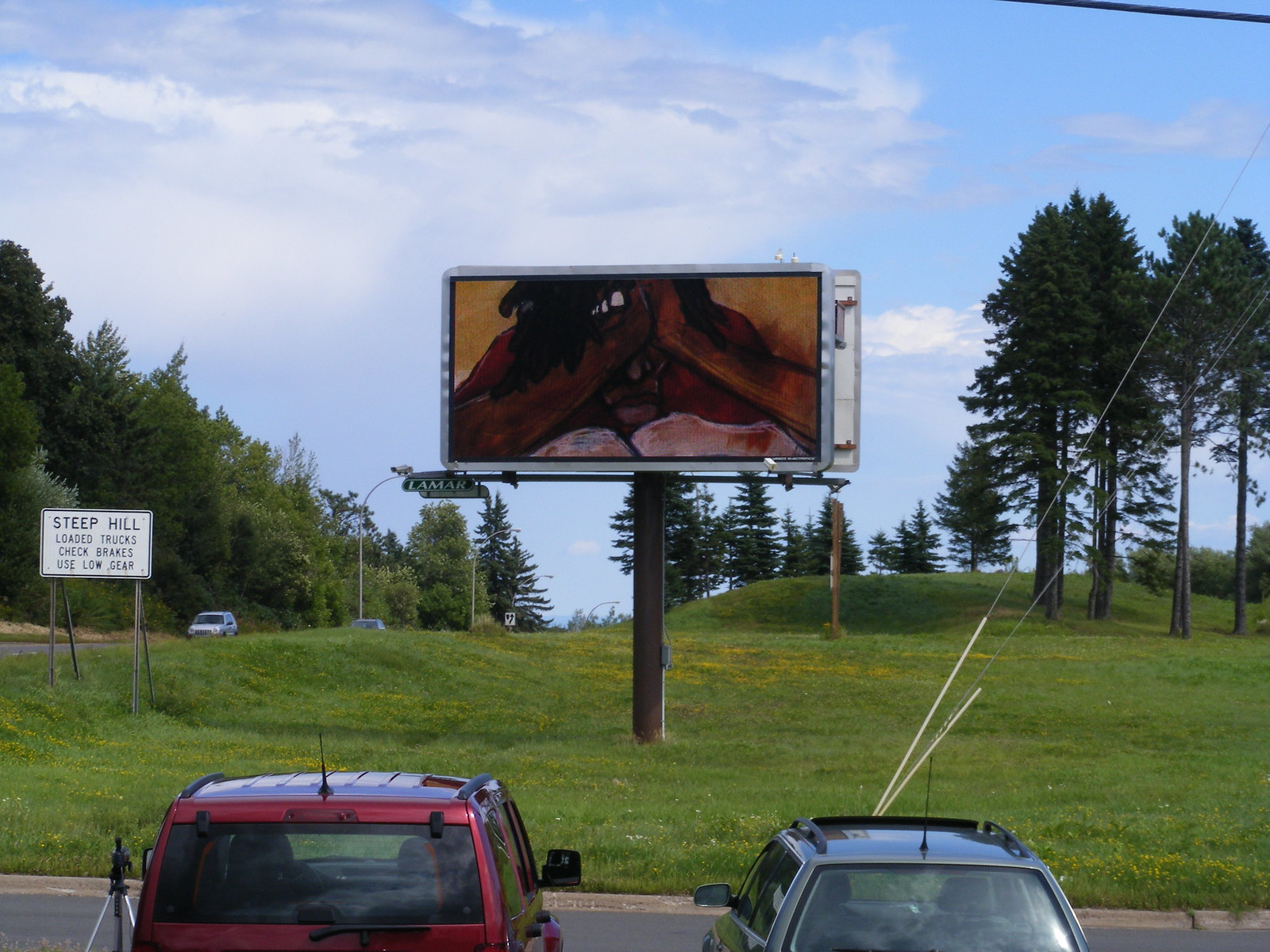A serene roadside parking lot stretches across the bottom of the photograph, where the tops of two cars are just visible. The parking lot is bordered by a verdant landscape, with lush grass and a line of trees that extend into the distance. Dominating the foreground is an unclear billboard, standing sentinel in front of the parked cars. From the left edge of the photograph, a road begins its journey, cutting through the scene and leading the eye towards the horizon. On the right side of the picture, a few cars travel down the road, adding a touch of life to the tranquil setting. Above, a vibrant blue sky is punctuated with fluffy white clouds, casting a soft light over the entire landscape.